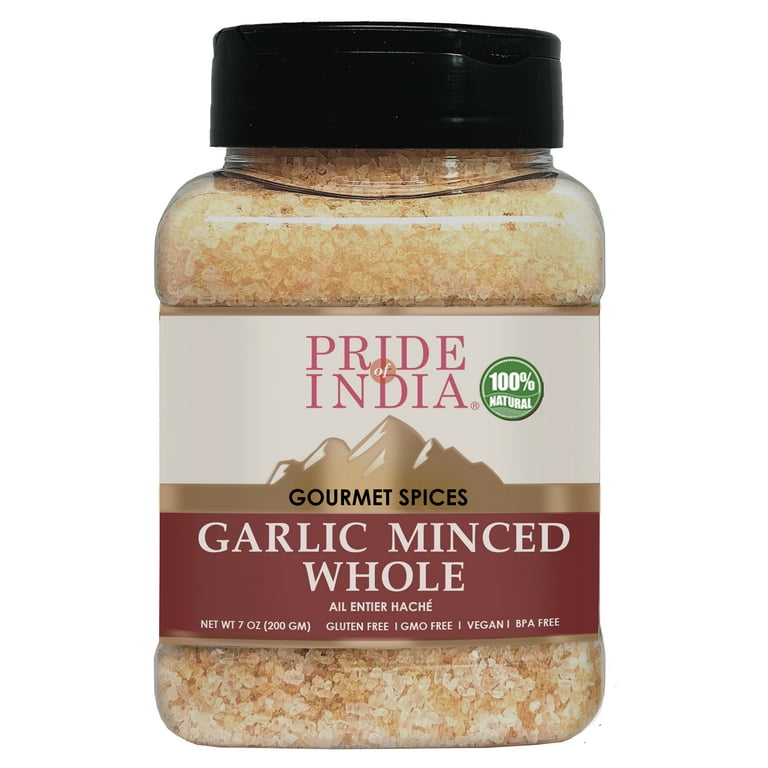This is a detailed close-up photograph of a clear, squarish plastic jar containing minced garlic. The jar, which has a black plastic lid, is filled with small, light yellowish-white chunks of garlic, visible through the transparent container. The product image is set against a sheer white background, highlighting the intricate details of the label.

The label itself is divided into three color sections: the upper part is a beige-gray, the middle features a brownish-gold band with a depiction of a mountain range, and the bottom section is a deep burgundy. At the top of the label, the brand name "Pride of India" is prominently displayed in a medium rose shade, accompanied by a green circle that reads "100% Natural." Below this, the text "Gourmet Spices" is written in black over the gold mountain range band. In larger white letters on the burgundy section, it states "Garlic Minced Whole." 

Additional details at the bottom of the label include "Net WT 7oz (200g)," along with indicators that the product is gluten-free, GMO-free, vegan, and BPA-free. This comprehensive presentation not only emphasizes the brand and product features but also ensures the health and safety information is clear and accessible.